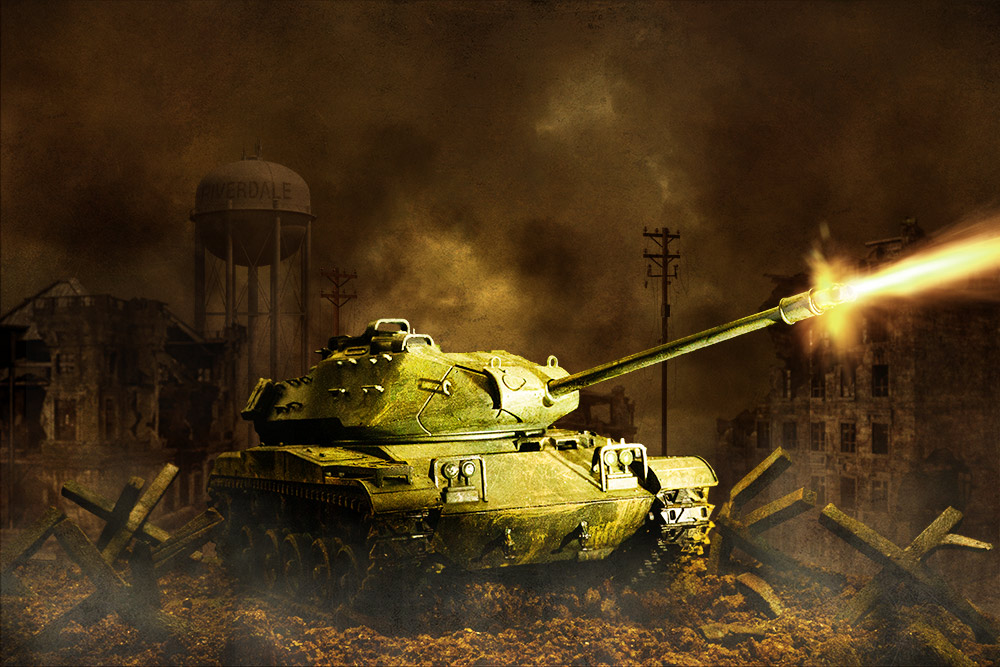The image appears to be a dark, ominous still from a video game, likely set in a war-torn, dystopian environment. Dominating the center is a prominently lit green tank, possibly an early Vietnam-era M1 type, firing its main gun towards the right. The sky is thick with dark clouds, smoke, and fog, enhancing the bleak atmosphere. Surrounding the tank is widespread wreckage, including dilapidated buildings, rubble, and debris. In the background, a water tower and an electrical pole stand amidst the ruins. On the left side of the image, there are several barricade jacks, reminiscent of those seen in modern conflict zones. The overall color palette is muted, with predominant shades of brown and black, contrasted only by the light green of the tank. There are no people present in this desolate scene, emphasizing the scale of destruction.